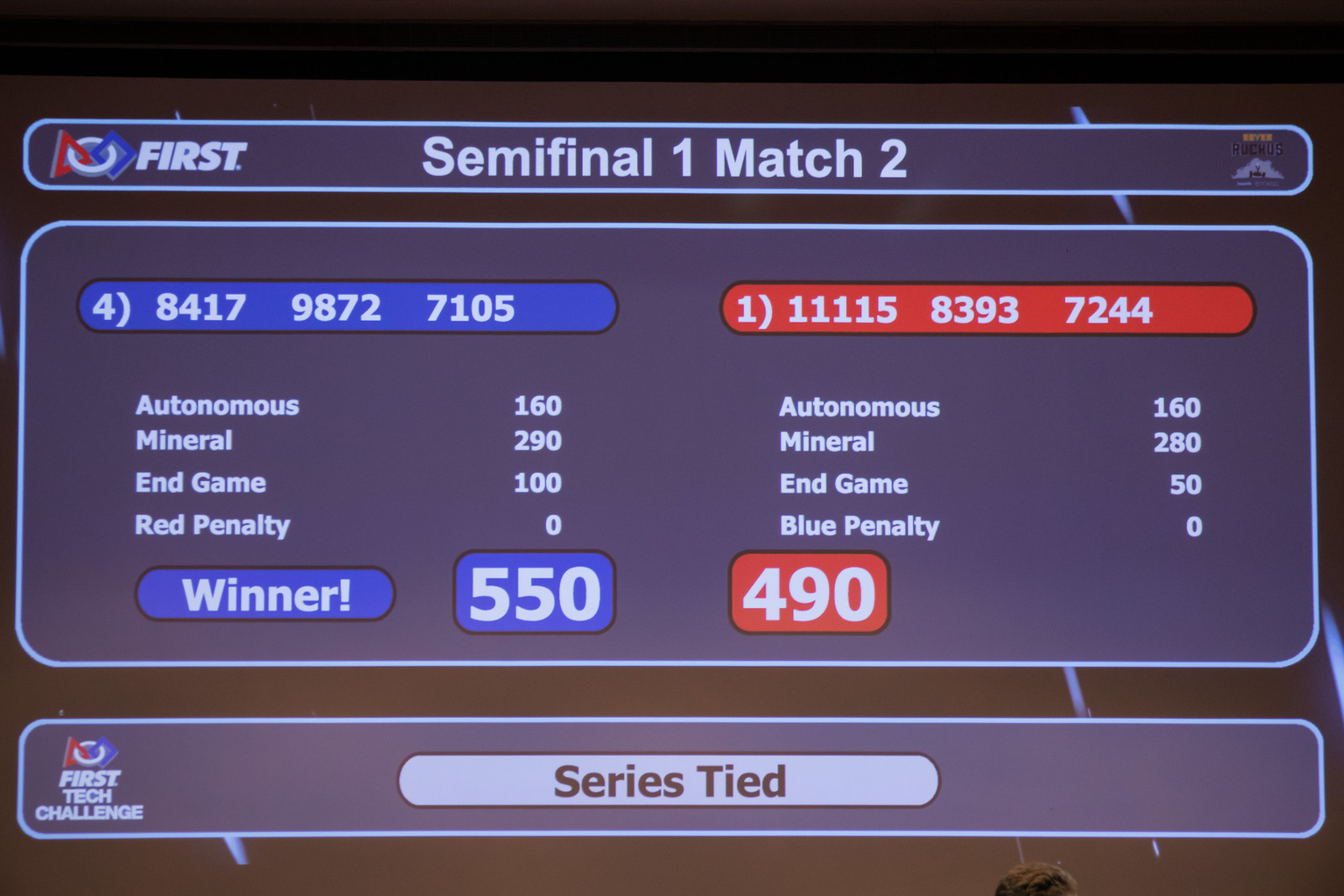The image depicts a game scoreboard from the First Tech Challenge semifinals, specifically Semi-Final One, Match Two. The header spans the top, featuring a blue background with a white font, and includes the event logo—an interlocked red triangle, blue square, and white circle. The primary section of the scoreboard is dominated by a large rectangular bubble with rounded edges, divided into two columns: one for the blue team and one for the red team. 

Each column starts with a header displaying a 12-digit number grouped in triplets, prefixed by a single-digit number within parentheses indicating a possible ranking. Beneath these headers, four lines break down the scores labeled "Autonomous," "Mineral," "Endgame," and "Red Penalty," each accompanied by specific numeric values.

The blue team's section concludes with a large blue banner proclaiming them the winner with a score of 550, while the red team shows a score of 490. At the very bottom, another bar indicates that the series is tied. The dominant color scheme includes shades of blue and red, with black borders and white text, giving the overall appearance a somewhat vintage feel, reminiscent of the 80s or 90s.